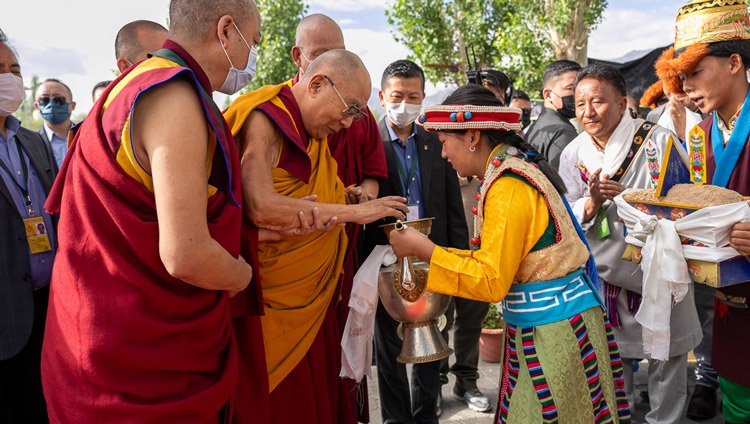This photograph captures a moment with the Dalai Lama, who is bald and wearing glasses, clad in traditional red and gold or yellow robes. He is surrounded by a diverse group of people, including several black-haired individuals and a few other monks. Central to the scene is a woman in traditional Tibetan or Indian attire, featuring a yellow blouse, muslin vest, hat, and skirt. She is holding a jug or pot out to the Dalai Lama, who appears to be placing his hand inside it. Behind her stands another man, holding a box full of rice. On one side, a cluster of Tibetan monks in mustard robes are interacting with the people, some of whom wear protective surgical masks. The setting is outdoors, with a visible sky dotted with white clouds and a couple of trees with green leaves, adding a serene, natural background to the scene.